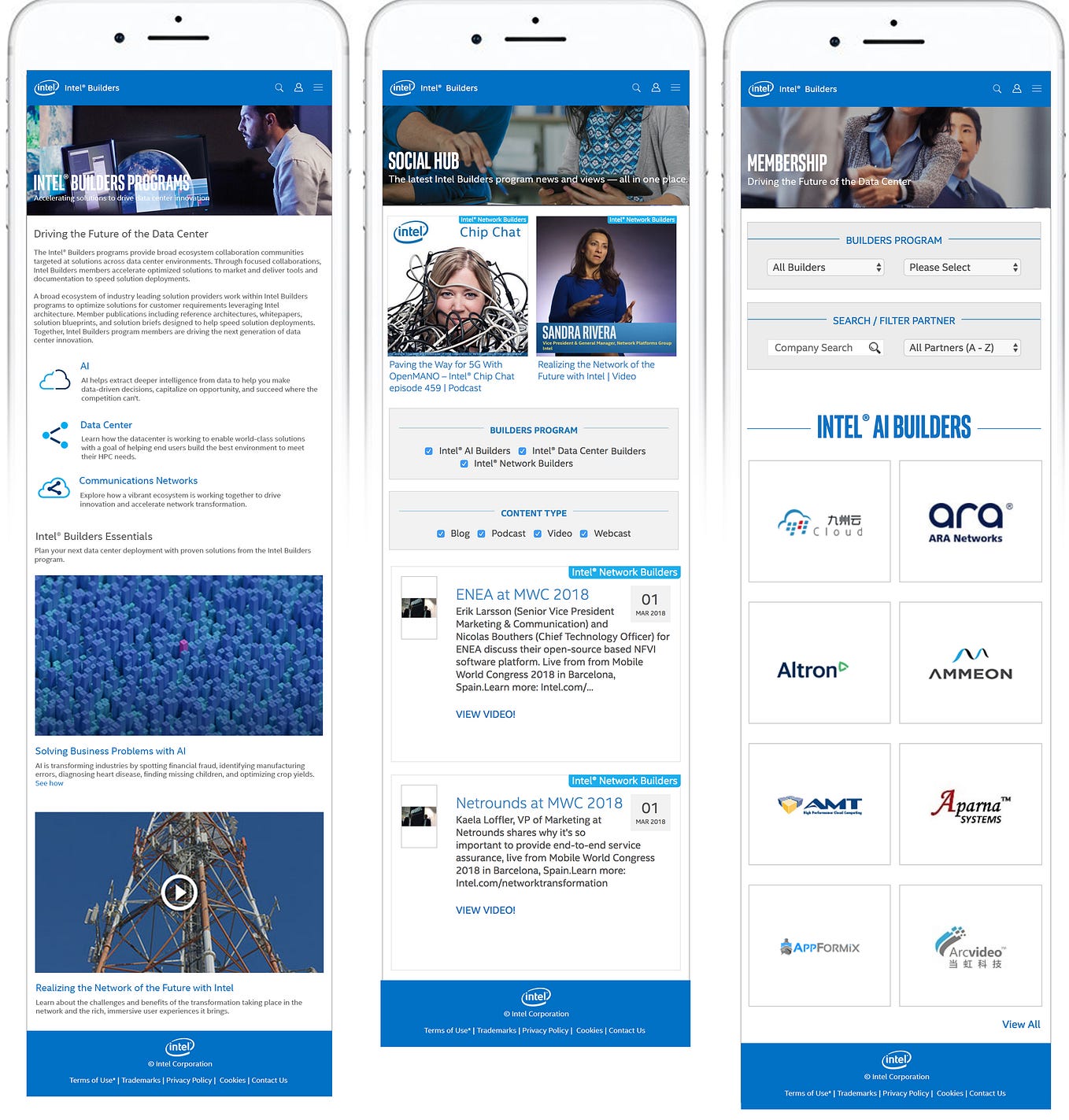This image is a row of three side-by-side screenshots of mobile devices, each displaying different sections of the Intel Builder's mobile site. 

- **Left Screenshot**: This screen captures the 'Intel Builder's Programs' page. At the top, there is a prominent white section with a header that reads, "Driving the Future of the Data Center," followed by two descriptive paragraphs and three bullet points. Below this text block, two large blue image links are displayed: the first directs to content about "Solving Business Problems with AI," and the second is a video with a blue background titled "Realizing the Network of the Future with Intel."

- **Center Screenshot**: This screenshot showcases the 'Social Hub' internal page of the Intel Builder's mobile site. The contents and specific features within this page are not detailed, but it is indicated as the main focus of this screen.

- **Right Screenshot**: Displayed here is the 'Membership' internal page, also part of the Intel Builder's mobile site. Similar to the middle screen, the exact details and features of this page are not elaborated upon in the provided description.

Each of the screenshots provides a glimpse into the different areas within the Intel Builder's suite of mobile web pages, emphasizing a cohesive theme centered around advancements and networking in technology.